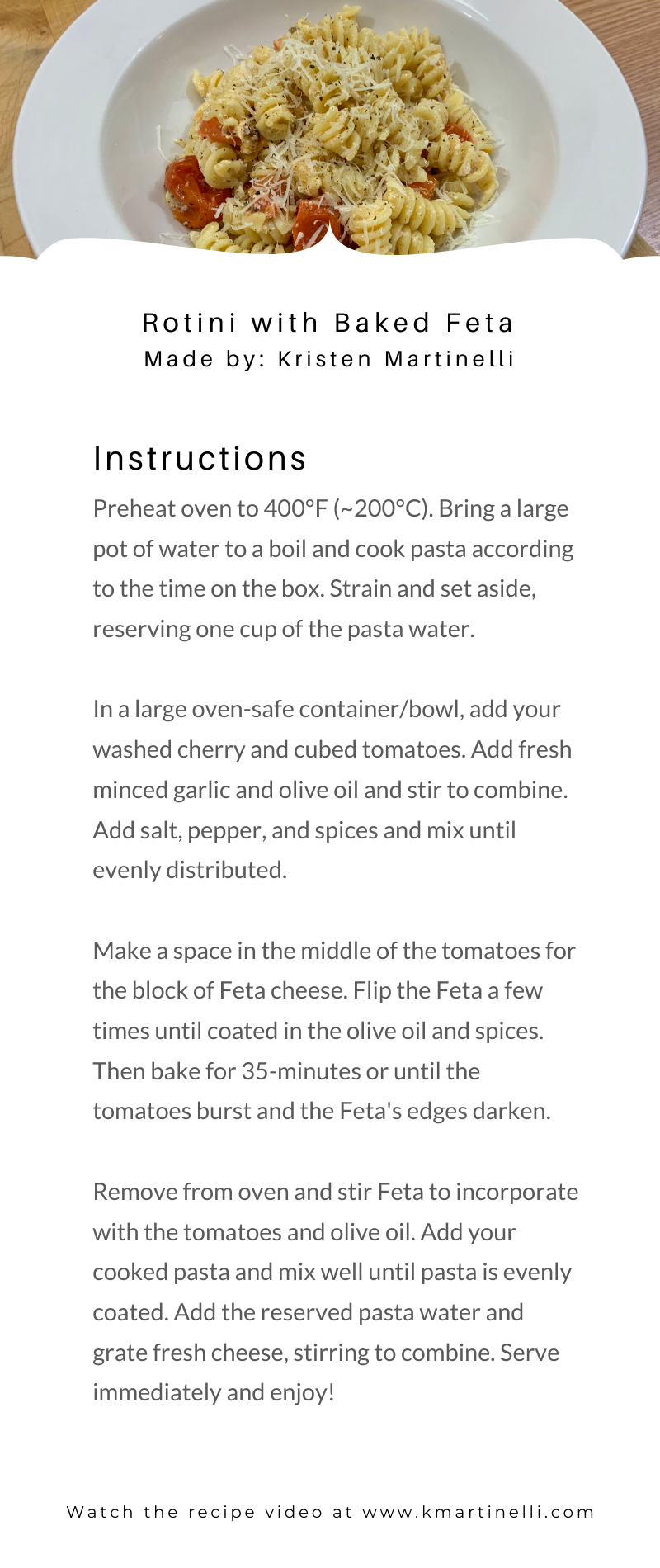Here's a refined and detailed caption for the image described:

---

**Screenshot of Food App Displaying Recipe Instructions**

The image is a screenshot of a food app's recipe page, focusing on a dish called "Rottini with Baked Feta" created by Kristen Martinelli. At the top of the page, there's an appetizing picture of the dish, featuring freshly cooked Rottini pasta in a wide-rimmed, almost bowl-like white plate set upon a rich brown wooden table. The pasta is artfully arranged and garnished, showcasing vibrant ingredients under natural lighting.

Just below the image, the recipe title "Rottini with Baked Feta by Kristen Martinelli" is prominently displayed. Following the title are the detailed cooking instructions set on a minimalist white background, ensuring readability.

In large, bold letters, the instructions begin with: 
- **Preheat oven to 400°F (approximately 200°C).**
- **Bring a large pot of water to a boil and cook the pasta according to the instructions on the box. Drain and set aside, reserving one cup of pasta water.**
- **In a large, oven-safe container, combine the cooked pasta, washed cherry tomatoes, cubed tomatoes, freshly minced garlic, and olive oil. Stir well.**
- **Season with salt, pepper, and your preferred spices, mixing until evenly distributed.**
- **Create a small space in the center for the block of feta cheese. Coat the feta with olive oil and spices by flipping it a few times.**
- **Bake for 35 minutes or until the tomatoes burst and the edges of the feta darken.**
- **Remove from the oven and stir to combine the baked feta with the tomatoes and olive oil. Add the cooked pasta and mix thoroughly until the pasta is evenly coated.**
- **Pour in the reserved pasta water and grate fresh cheese on top, stirring to combine.**
- **Serve immediately and enjoy!**

At the bottom edge of the picture, elegant, symmetrical flourishes add a decorative touch to the page. To further enhance the cooking experience, viewers are invited to watch the recipe video at **www.kmartinelli.com**.

---